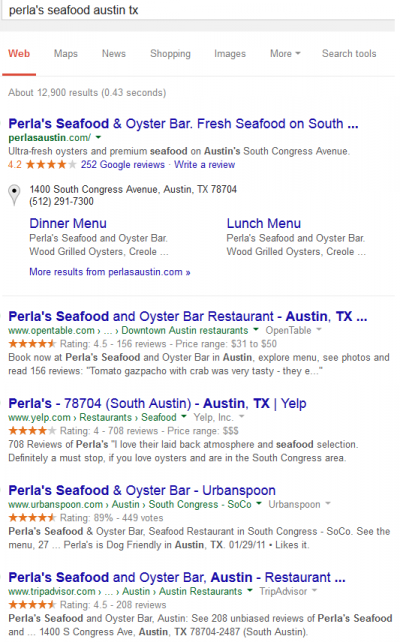This is a Google search result page for Perla's Seafood in Austin, Texas, displaying approximately 12,900 results. The top entry is Perla's Seafood and Oyster Bar, located on Austin's South Congress Avenue, boasting a rating of 4.2 stars from 252 Google reviews. The listing provides options to rate or review the restaurant, along with insets for the map location, dinner menu, and lunch menu. Subsequent search results reflect similar information sourced from platforms such as OpenTable, Yelp, Urban Spoon, and TripAdvisor. On Yelp, Perla's Seafood has garnered 708 reviews, underscoring its popularity and high ratings—4.5 stars, 4 stars, and 89%, respectively. These entries appear to be organic results rather than paid advertisements. The search results likely come from a mobile device, though it could also be from a computer.